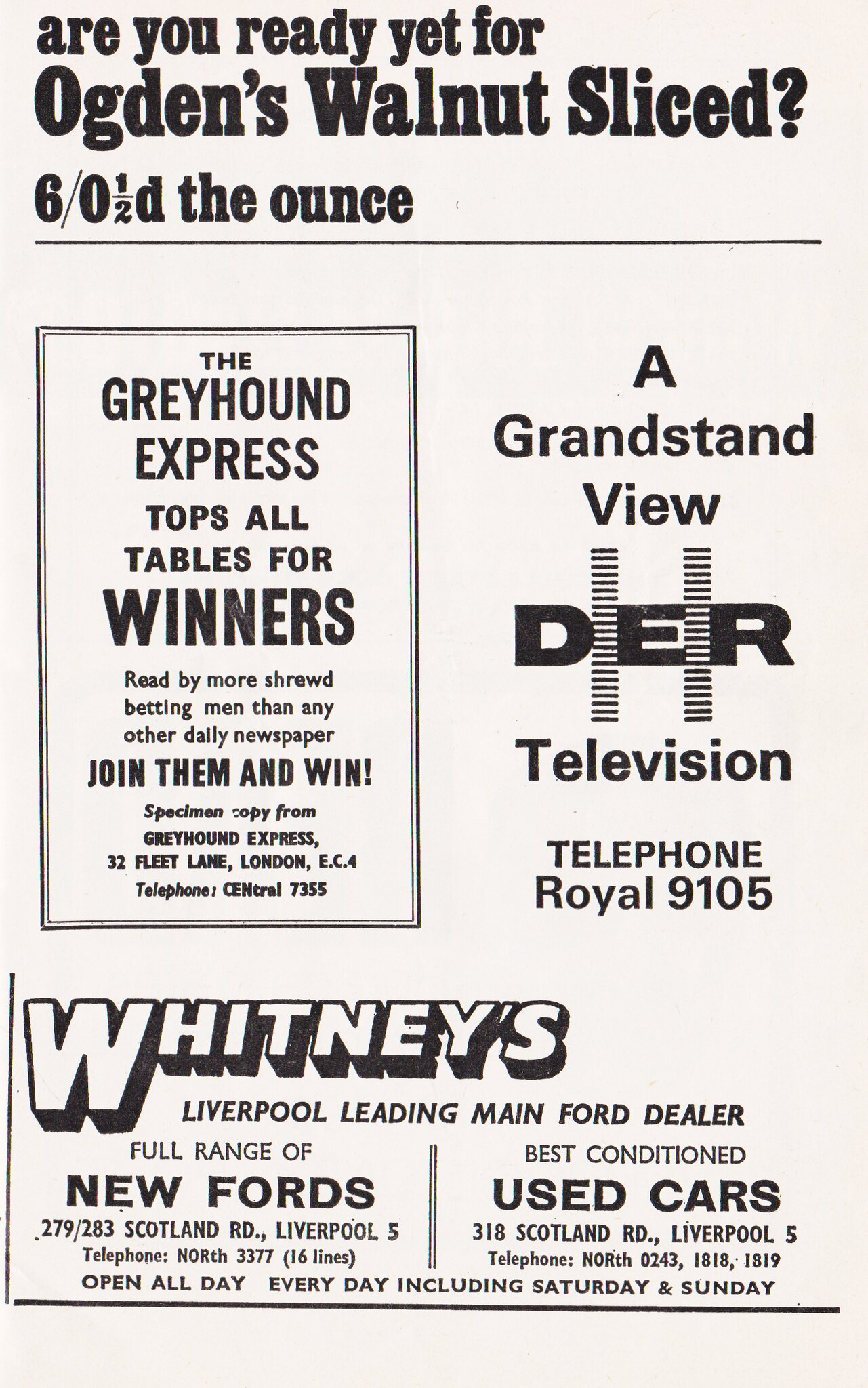This image depicts what seems to be an advertisement clip, potentially cut out from a classifieds section or a newspaper, on a gray background. At the top, in bold black letters, it reads, "Are you ready yet for Ogden's Walnut Slice?" Below this, there's a notation, "6/0, 1/2 D the ounce," followed by a long horizontal divider. On the left side, there is a box that includes promotional text for the "Greyhound Express," which claims to top all tables for winners and is read by more shrewd betting men than any other daily newspaper. It invites readers to "Join them and win!" and provides contact information: "Specimen copy from Greyhound Express, 32 Fleet Lane, London EC4," and telephone number "CENTRAL 7355."

Adjacent to this box, it reads, "A grandstand view," followed by "DER television," and "Telephone Royal 9105." At the bottom, in striking 3D print, it displays "Whitney's" with white letters against a black shadow background. This part highlights "Liverpool Leading Main Ford Dealer," offering a full range of new Fords at "279/283 Scotland Road, Liverpool 5," with the telephone number "North 3377 (16 lines)." The advertisement also features "Best Condition Used Cars" located at "318 Scotland Road, Liverpool 5," with the contact numbers "North 0243 1818 1819." At the very bottom, it notes, "Open all day, every day, including Saturday and Sunday."